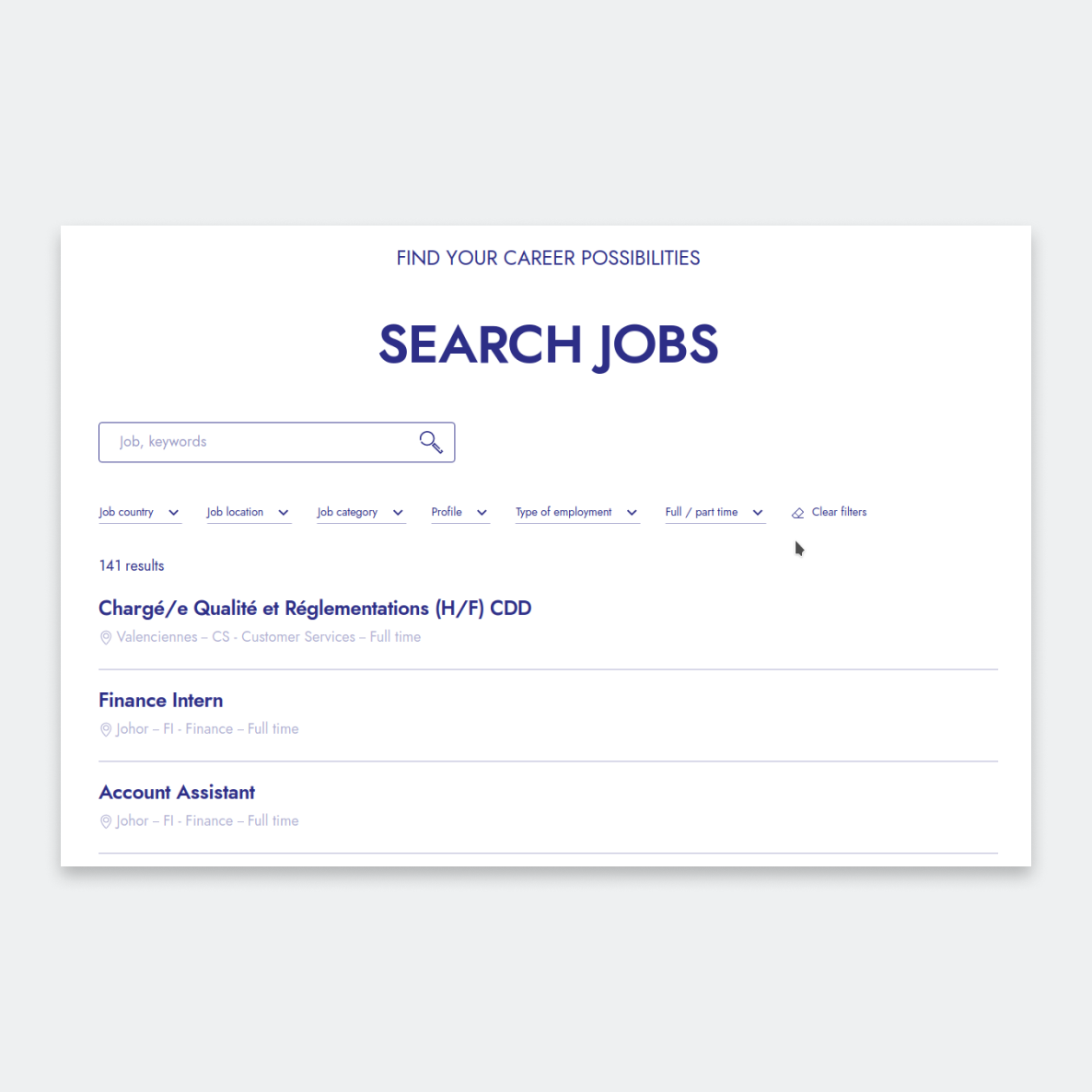In the foreground of the image, a bright white box stands out against a slightly dimmer white background. At the top center inside the box, the text "Find Your Career Possibilities" is prominently displayed in blue. Directly below this, in bold blue letters, reads "Search Jobs." 

On the upper left corner below the bold text, there is a blue-highlighted search bar with placeholder text in gray that reads "job, keywords." To the right of the search bar, a blue magnifying glass icon signifies the search function.

Below the search bar, a set of filter options is presented. From left to right, these include:
- "Job Country" with a drop-down arrow
- "Job Location" with a drop-down arrow
- "Job Category" with a drop-down arrow
- "Profile" with a drop-down arrow
- "Type of Employment" with a drop-down arrow
- "Full/Part-Time" with a drop-down arrow 

Beside these filters, there is an eraser icon followed by the text "Clear Filters" in blue.

Beneath the filter options, on the left side, "141 Results" is clearly displayed. On the right side, there is a black cursor arrow icon. 

The job listings start below this section, the first listed job being "141 results" in blue. The subsequent job titles are listed as follows:
- "Chargé/Chargée de Qualité et Réglementations (H/F)" marked with a blue font, identified by the accented characters indicating it’s in French, and followed by the term "CDD".
- "Finance Intern" displayed in blue underneath the French job title.
- "Account Assistant" also in blue, appearing just below the "Finance Intern" listing.